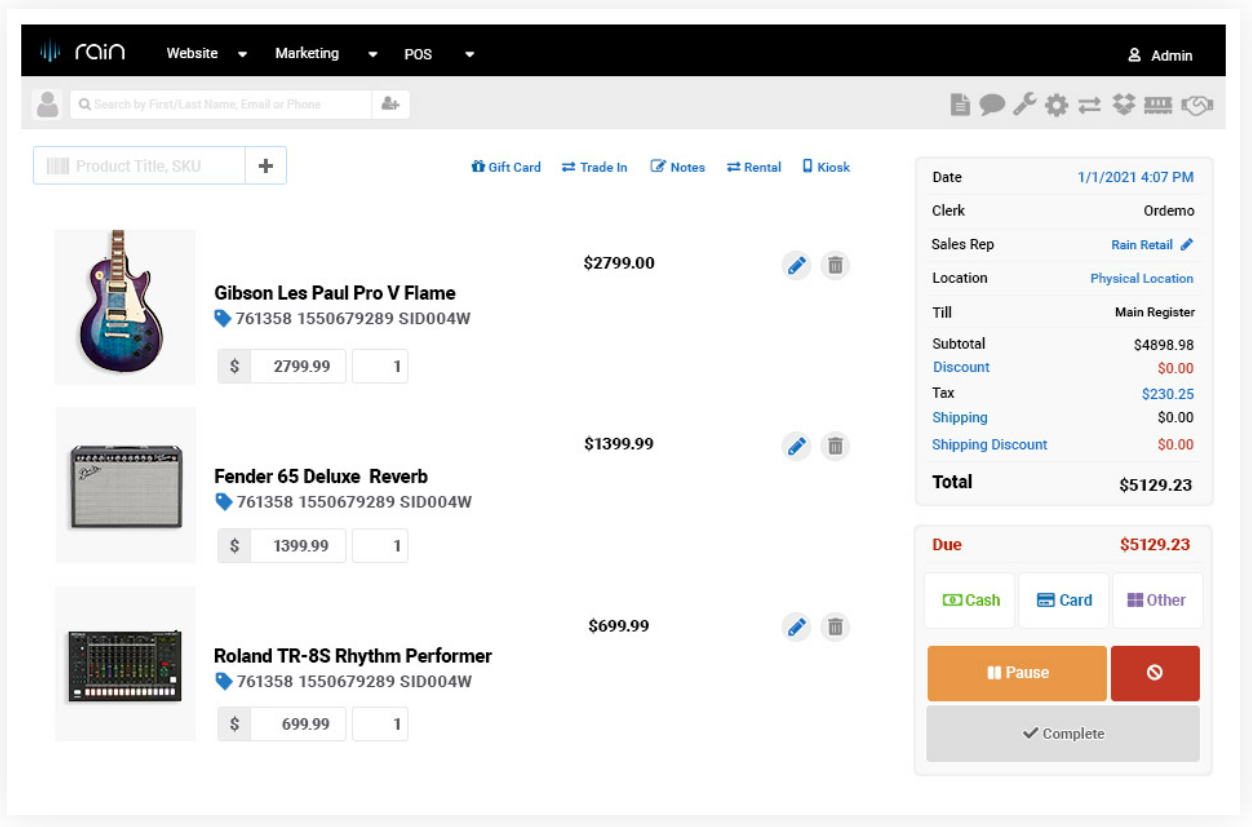The webpage, named "Rain" in lowercase white letters against a black top header, serves as an online storefront for musical equipment. The blue Rain logo, resembling a waveform, is situated to the left of the store name. The site features a minimalist design with the majority of the page in white backdrop and black text descriptions.

Highlighted items for sale include a striking blue guitar, a grey reverb amplifier, and a Roland TR-8S Rhythm Performer, a sophisticated mixer designed for combining various audio elements. 

The header beneath the main header is grey, complementing the simple aesthetic, with light blue fonts used for additional sections and features of the website. Various functional buttons in blue, including an "Edit" button next to each item, allow users to modify their selections.

Key sections such as Gift Card, Trade-In, Notes, Rental, and Kiosk are denoted with blue text, offering a range of service options. The totals section, meticulously detailed, breaks down item prices, discounts, taxes, and shipping costs. Payment options, including cash, card, and others, are displayed below the totals, alongside operational buttons like a pause and a red stop button, facilitating the ordering process.

Overall, the webpage is clean and user-friendly, providing detailed sections for an efficient shopping experience for musical enthusiasts.